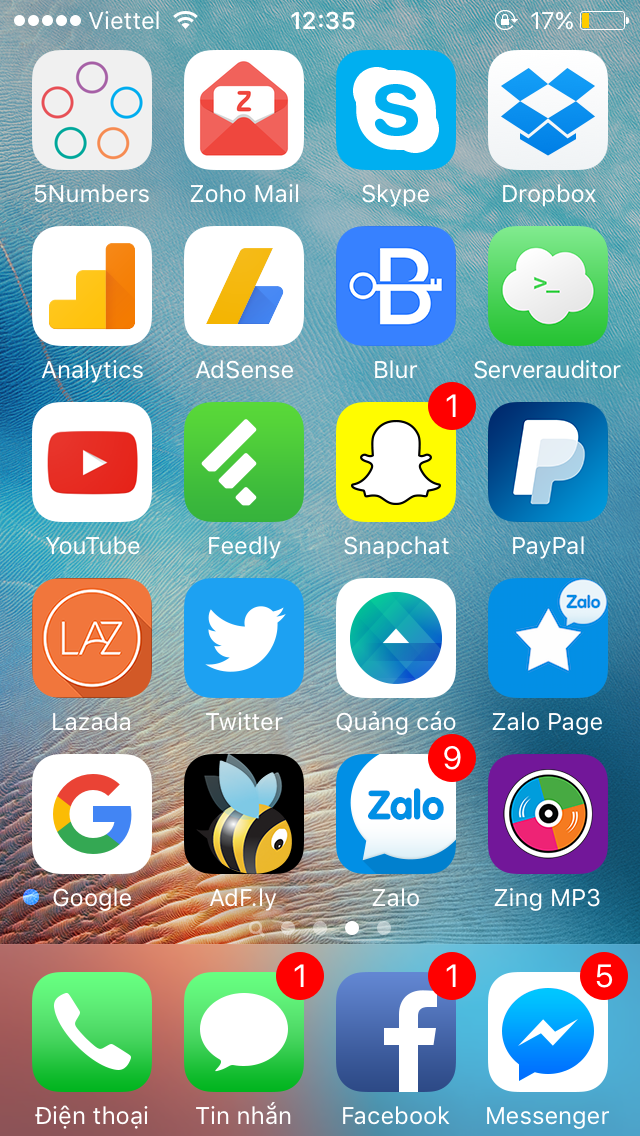The image depicts the home screen of a heavily utilized smartphone belonging to an individual who appears to rely heavily on mobile communication. The screen is cluttered with numerous application icons, each representing different tools and platforms the user frequently engages with. Among these, standard apps like the phone dialer are present, but there are also many social media and messaging apps prominently displayed.

Clusters of red notification badges indicate the user has multiple unread messages, suggesting a high level of social interaction. Apps such as Snapchat, Zalo, and WhatsApp are visible, as is the Facebook app along with its Messenger counterpart. The presence of so many unread notifications underscores the individual's proactive use of these platforms for staying in touch with contacts.

The status bar at the top reveals the phone's service provider is Viettel, a telecommunications company, which points towards a Vietnamese context as Viettel is a major network in Vietnam. The time on the phone is 12:35, and the battery level is critically low at 17%, indicating the device needs charging soon to avoid shutting down.

The home screen is entirely filled with icons, leaving no empty space, which may imply the user has a broad range of interests and activities that require a variety of applications. Furthermore, icons with text possibly in Vietnamese support the likelihood that the user is operating in a Vietnamese linguistic landscape, reinforced by the choice of local service provider Viettel. This meticulous arrangement of apps suggests that mobile communication is a pivotal aspect of the user’s daily routine.